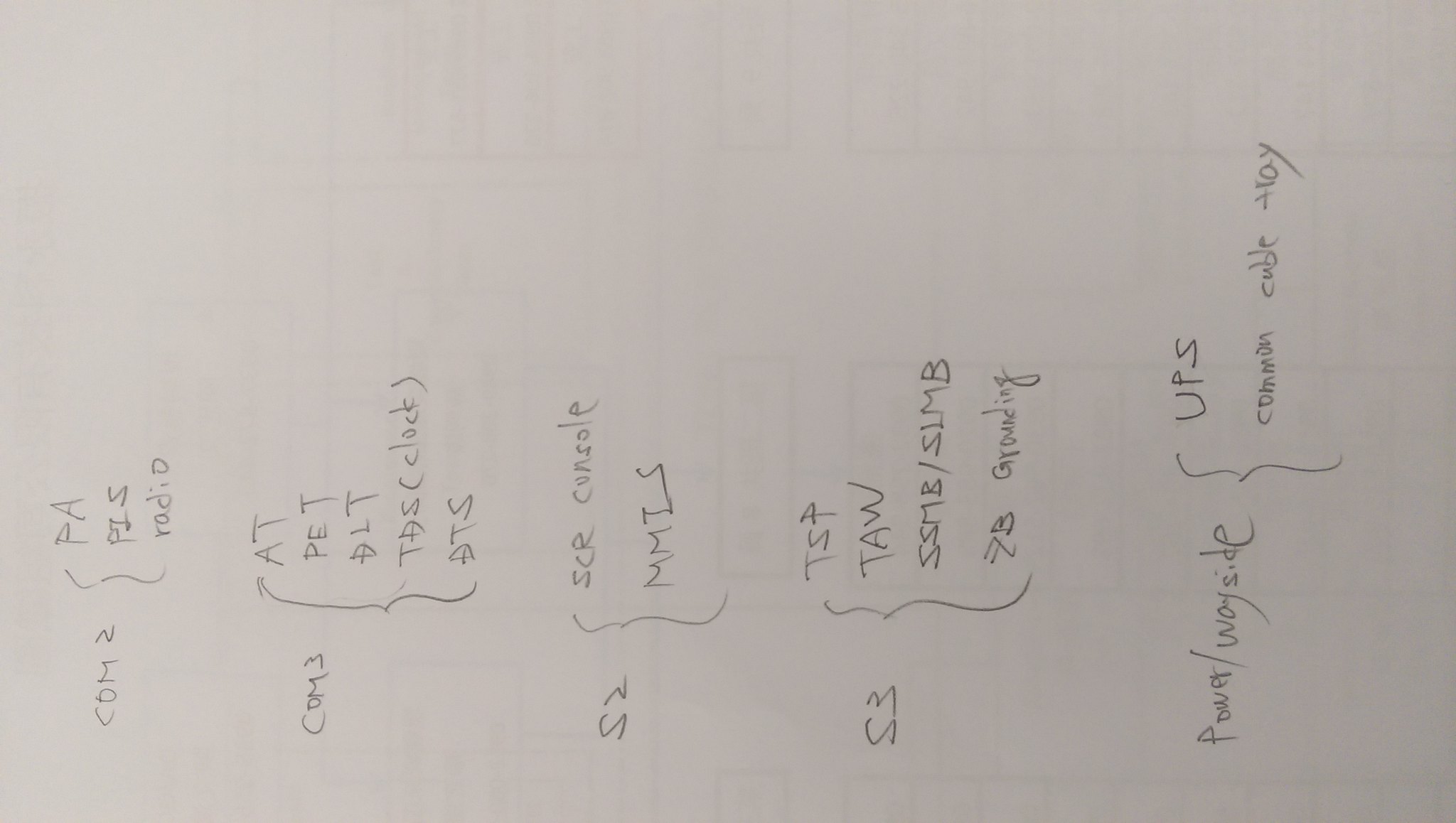The image displays a white piece of paper oriented horizontally. It contains five distinct sections of handwritten text:

1. The first section starts with "COM2 (P-A)" followed by lowercase letters "p-z-s" underneath. Below that is "R-O-DI" with a capital "D".

2. The second section reads "COMCOM3", accompanied by a bracket on the right. At the top of this section, it lists "A-T" followed by "P-E-T" underneath. Below that is a triangle with a horizontal line through it, then "L-T". The next line contains "T-A-S-C(CLOCK)" in capital letters, and the final line has an arrow pointing right with "T-S".

3. The third section, labeled "S-T", includes a bracket to the right with "S-C-R" and the word "CONSOLE". Below that are capital letters "M-M-T-S".

4. The fourth section, denoted "S-3", displays "T-S-P", "T-A-W", and "S-S-M-B/S-I-M-B". Additionally, there is an arrow pointing towards a "B" and the word "GROUNDING".

5. At the bottom of the paper, it says "POWER/WAYSIDE" next to a bracket with "UPS", followed by "COMMON CUBE ALLOY".

This detailed layout suggests a structured and organized set of instructions or information, likely related to a technical or engineering field.